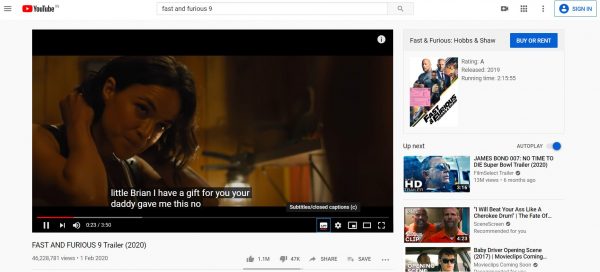Screenshot of a Cropped YouTube Home Page Featuring Fast and Furious 9 Trailer

The screenshot captures a cropped view of the YouTube home page. At the top of the page, the familiar YouTube logo is prominently displayed. On the left side of the logo is the menu icon. Centrally placed at the top is the search bar, with "fast and furious 9" typed in lowercase letters. On the right side of the search bar are a series of icons: the video upload icon, the view toggle icon, a three-dot menu, and finally, the sign-in button found on the far right.

The background of the page is a muted gray. On the left side, a large video player takes up significant space, showcasing a scene from the "Fast and Furious 9" trailer, complete with subtitles. Directly below this player, the video title "Fast and Furious 9 trailer (2020)" is displayed, followed by information about the number of views and the upload date.

In the lower section of the video player on the left, you can find various interactive elements: the number of likes, the number of dislikes, and icons for sharing and saving the video.

On the right side of the screen, at the top, there is an advertisement for "Fast and Furious: Hobbs and Shaw," offering options to buy or rent the movie. Below this ad, the section labeled "Up next" is visible, featuring the "Autoplay" toggle, which is currently switched on. Beneath this, a vertical list of suggested videos for the viewer to watch next is displayed.